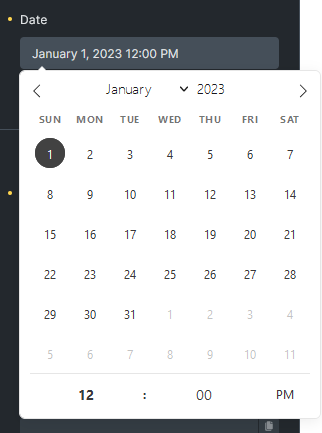This image is a cropped screenshot from a smartphone, focusing on the calendar interface. The background at the top of the screen is black with a small white text indicating the word "Date," accompanied by a yellow dot on its left. Centered below this, there is a grey box displaying the date and time as "January 1st, 2023, 12pm." This grey box has an expandable drop-down menu beneath it.

The drop-down box highlights various elements: at the top, navigation arrows appear on either side to scroll through the months, and below the year, a downward arrow allows for year adjustment. The days of the week—Sunday through Saturday—are listed horizontally across the top of the box.

The specific date is marked: January 1st is enclosed in a black circle, indicating it is a Sunday and the date selected. This selected date, "January 1st, 2023, 12pm," is reflected back in the grey box at the top of the drop-down menu, confirming the chosen date and time.